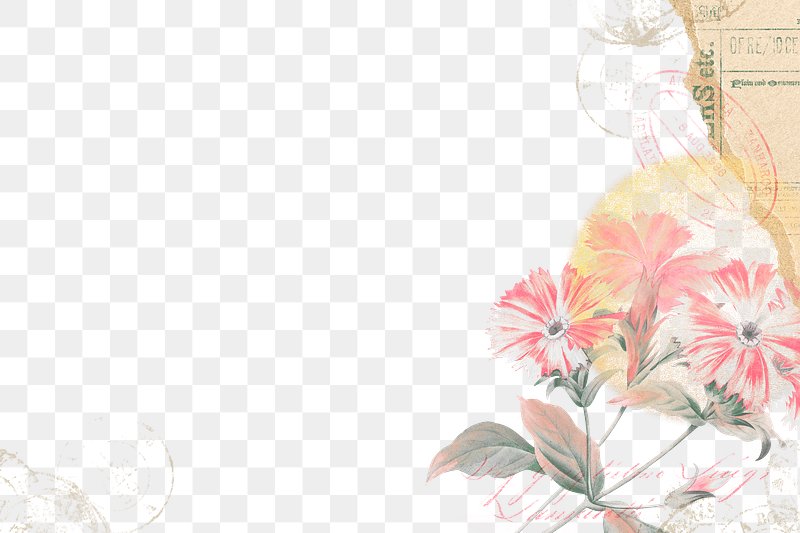The image depicts a graphic illustration resembling a vintage postcard, dominated by a checkerboard pattern composed of gray and white squares, leaving a clear transparent background on the majority of the left side. The right section prominently features a floral motif with delicate flowers displaying thin, ragged pink petals, accompanied by green leaves with subtle pink tones. Notably, the bottom right corner showcases a cluster of these flowers. Stems are thin, adding to the delicate feel of the artwork.

In the upper right corner, there appears to be a torn section of an envelope, adorned with green letters that are partially legible, hinting at postal service usage. This part of the illustration also contains postmark-like stamps, contributing to the vintage aura. A yellowish water stain extends from the torn edge into the floral design, blending the elements. Additionally, similar postal marks can be found in the left-hand corner of the image.

The floral arrangement occupies roughly 14 columns from the right end of the checkerboard pattern, which consists of 20 rows in total, though the first row is slightly cut off at the bottom. The detailed composition tethers the modern graphic style with nostalgic elements, making it a unique piece of digital art.